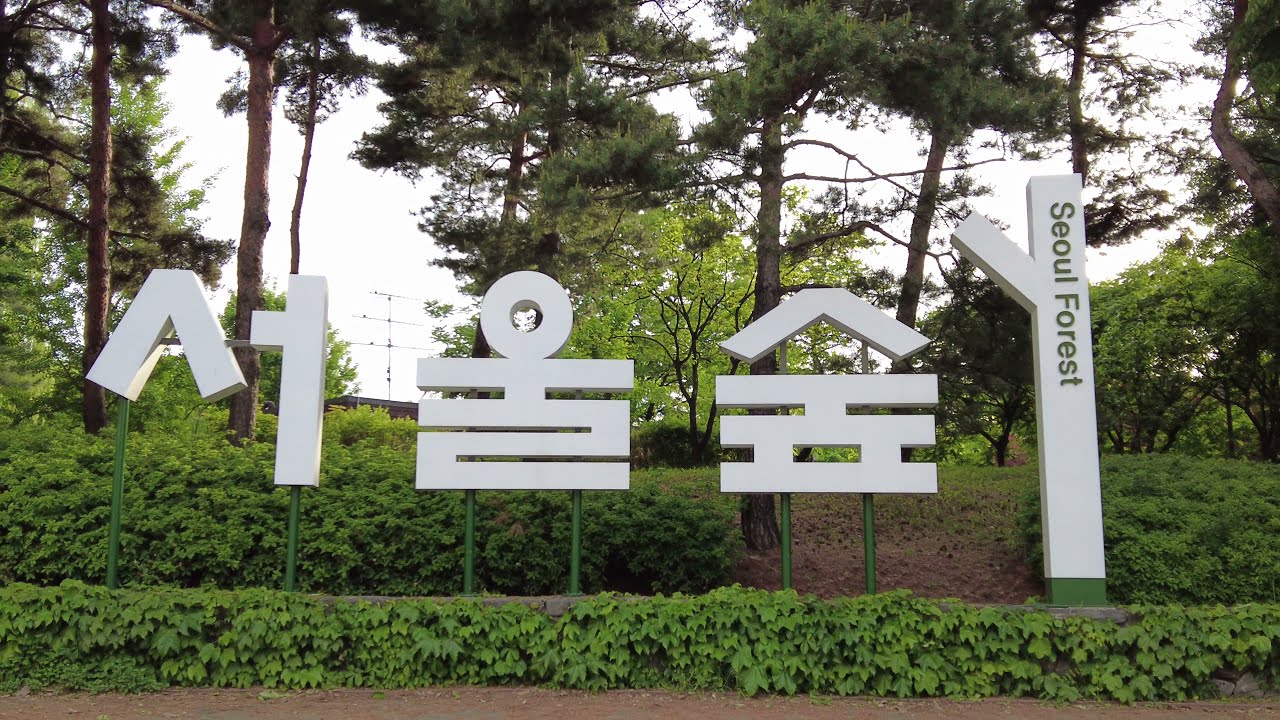The image is a color photograph in landscape orientation, depicting a meticulously maintained forest setting. The forest features sparsely spaced trees, approximately 10 feet apart, predominantly composed of tall, slender pine trees with barren trunks and dense, green tops. Central to the image is a set of five wooden signs, painted white and inscribed with Korean characters, standing on metal poles about three feet tall. The arrangement includes a vertical white post on the far right, extending at a 45-degree angle near the top, emblazoned with the words "Seoul Forest" in both uppercase and lowercase letters. The signage is situated on a gently sloping hillside lush with green ivy that extends to the forest floor, suggesting an inviting natural setting promoted by the signs. The overall style of the photograph is realistic, capturing the serene and organized beauty of the forest in vivid detail.